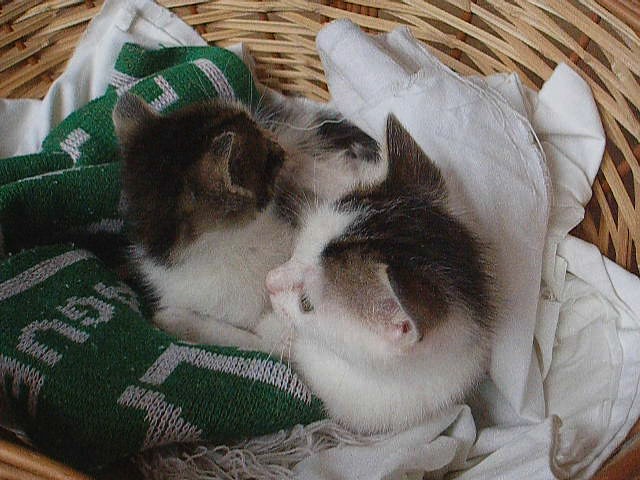The image is a close-up photograph of two juvenile kittens nestled together in a light tan wicker basket. They are lying on a combination of blankets—one prominently green with some white stitch work and lettering, and another purely white. The kittens, mostly white in color, have dark brown markings on their heads and ears, which add to their distinct appearance. The kitten at the front, with a little pink nose and brown ears, looks off to the side, revealing a big brown spot that covers both ears and part of its head. The other kitten, slightly behind and appearing to hug its sibling, faces away, showing a white chest and a mostly brown head. The serene scene suggests they are resting peacefully in their snug, blanket-filled basket.